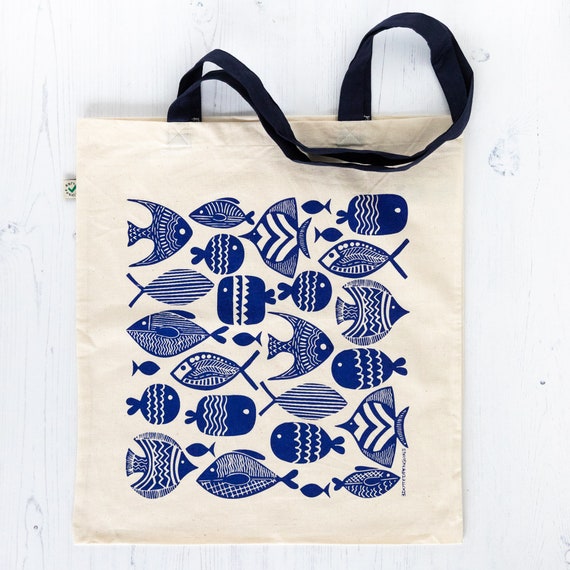This is a photograph of a square, cream-colored canvas tote bag adorned with various stylized, blue fish illustrations. The fish artwork is two-dimensional and flat, showcasing a range of designs from simplified shapes with minimal features like dots for eyes and small fins, to more intricate textures with ridges and lines, both straight and wavy. Some fish appear realistic, while others are more abstract. The bag features two black straps for handles, suitable for carrying over the shoulder, making it ideal for uses such as grocery shopping or a summer beach outing. There's also a small tab on the side with a green check mark. The bag is resting on, or possibly hanging against, a white, wood grain background.